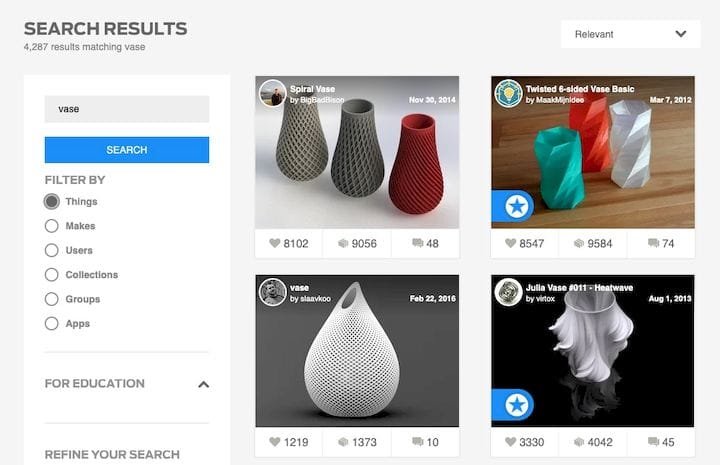**Search Results Page for "Vase"**

- **Total Results:** 4,287 results matching "Vase".
- **Sorting Options:** A drop-down box on the right side allows sorting by "Relevance".
- **Search and Filter Options:** A blue search button is present along with filter options labeled "Files," "Makes," "Users," "Collections," "Groups," "Apps." The filters are highlighted, and there is an option to "Refine Your Search."

**Displayed Vases:**

1. **Spiral Vase**
   - **Creator:** Big Bad Reason
   - **Date:** November 20, 2014
   - **Likes:** 8,102
   - **Comments:** 48
   - **Others:** 9,056 (icon not identified)
   - **Description:** This vase features a geometric honeycomb, diamond-like pattern.

2. **Twisted Six-Side Vase Basic**
   - **Date:** March 7, 2012
   - **Likes:** 8,547
   - **Comments:** 74
   - **Others:** 9,584 (icon not identified)
   - **Description:** This vase has a twisted, threaded design.

3. **Vase**
   - **Date:** February 22, 2016
   - **Likes:** 1,219
   - **Comments:** 10
   - **Others:** 1,373 (icon not identified)
   - **Description:** A basic white vase with a teardrop shape.

4. **Julia Vase**
   - **Title:** Number 9, Heat Wave
   - **Date:** August 1, 2013
   - **Likes:** 3,330
   - **Comments:** 45
   - **Others:** 4,042 (icon not identified)
   - **Description:** This vase resembles a plume of smoke.